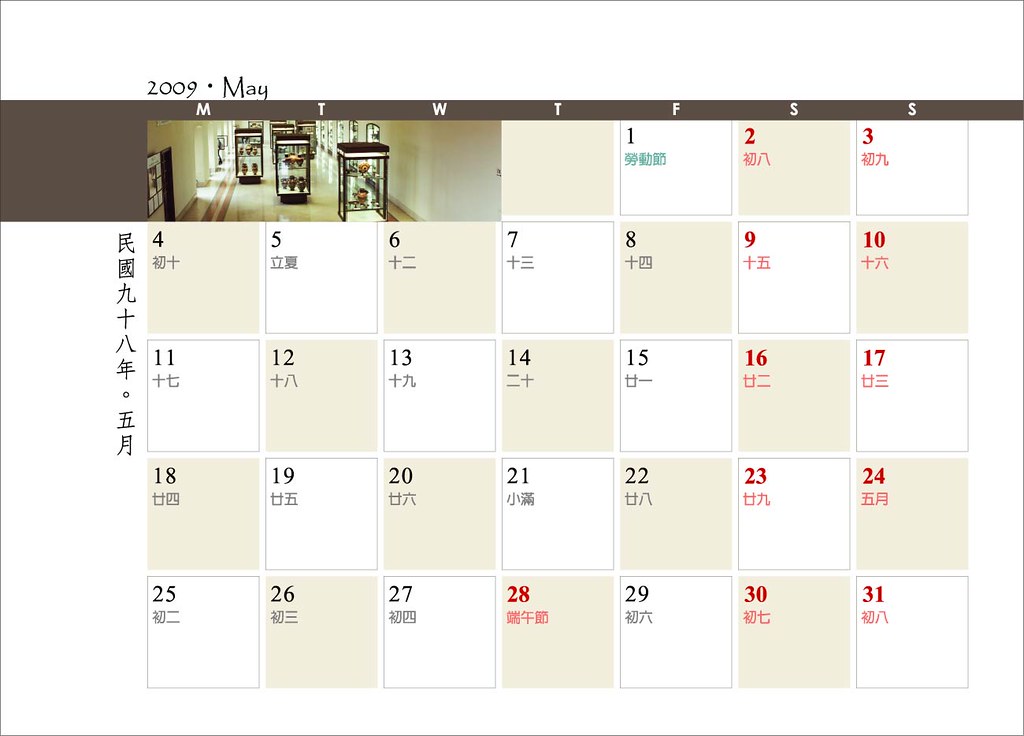This image depicts a page from a Chinese-inspired calendar for May 2009. The calendar features a checkerboard design with alternating cream and white squares. The days of the week are labeled with numbers in the top left corner of each square: weekdays in black and weekends in red, including the 28th. Each date is accompanied by a corresponding Chinese character beneath the number.

Notably, the top section of the calendar features a photograph spread across the first three days of the month, Monday through Wednesday, showing what appears to be glass jewelry cases or display cases containing valuable items. Along the left side, a vertical column of Chinese characters provides additional cultural context.

Overall, the calendar maintains a harmonious blend of traditional Chinese aesthetics and functional design, with an emphasis on the alternating square color scheme and bilingual day labels.